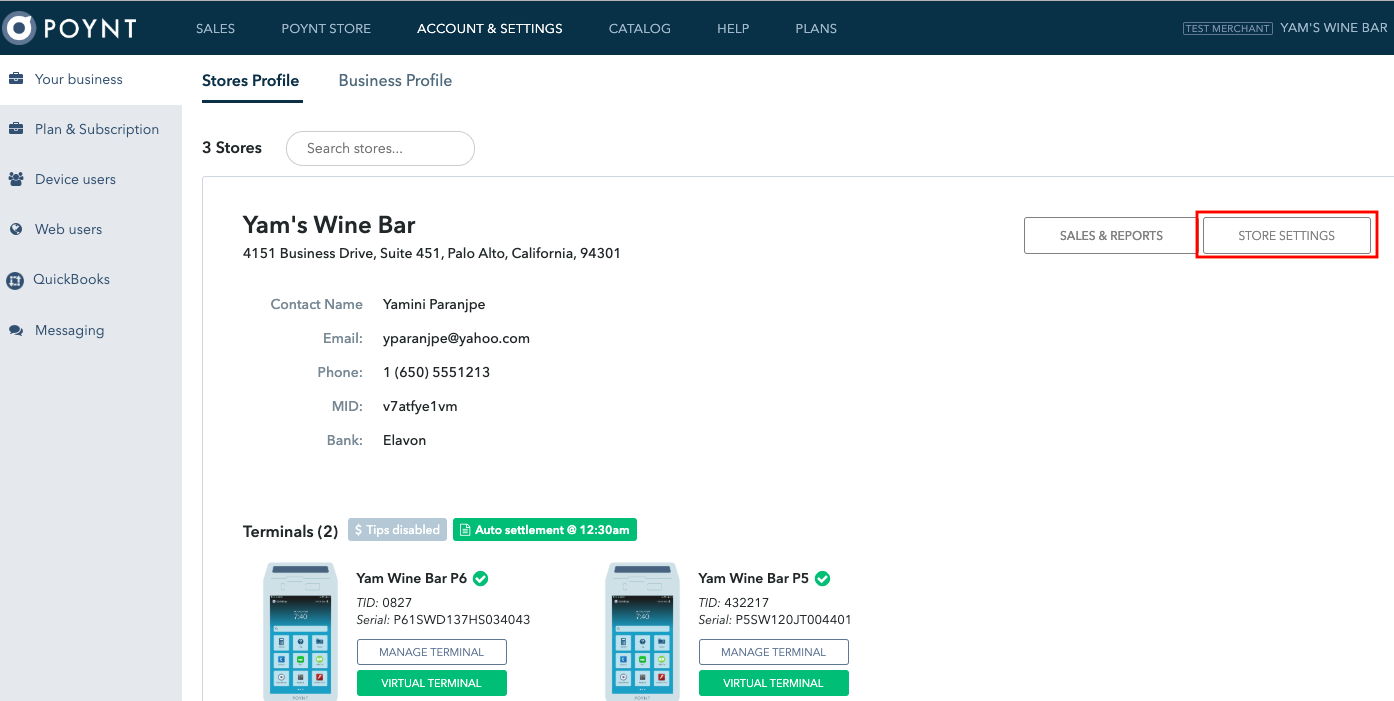The top of the website features a distinctive dovetail-patterned border in color. On the left-hand side, against a white background, the word "POYNT" is prominently displayed in all capital letters, suggesting the name is "Point" but with a unique spelling. 

To the right, there's a category menu with items such as "Sales," "Point Store," "Accounts," and "Settings" appearing in a bolder, brighter white, indicating the currently active area. Other menu items in this section include "Category," "Help," and "Plant." Below this menu, the screen displays the labels "Test Merchant" and "Yams and Wine Bar."

The main content area transitions to a clean white background. In the middle, taking up more space, is the store's profile section, with the heading "Store's Profile" in dark blue and underlined, indicating a clickable link. Beneath that is "Business Profile," shown in gray, suggesting the current section is "Store's Profile."

Further down, there is a subheading in light gray that reads "Three Stores," accompanied by an outlined oval featuring the placeholder text "Search Stores..." The primary store displayed is "Yams Wine Bar" in bold black text. Detailed information listed includes:

- **Address:** 4151 Business Drive, Suite 451, Palo Alto, California, 94301
- **Contact Name:** Yemini Paranjpe
- **Email:** yparanjpe@yahoo.com
- **Phone:** (650) 555-1213
- **MID (Merchant Identification):** V7ATFYEV1VM
- **Bank:** Elavon
- **Terminals:** Yams Wine Bar 6 with virtual terminal options listed as two terminal virtual options. 

This comprehensive layout provides an efficient and detailed overview of a store's profile and associated details.